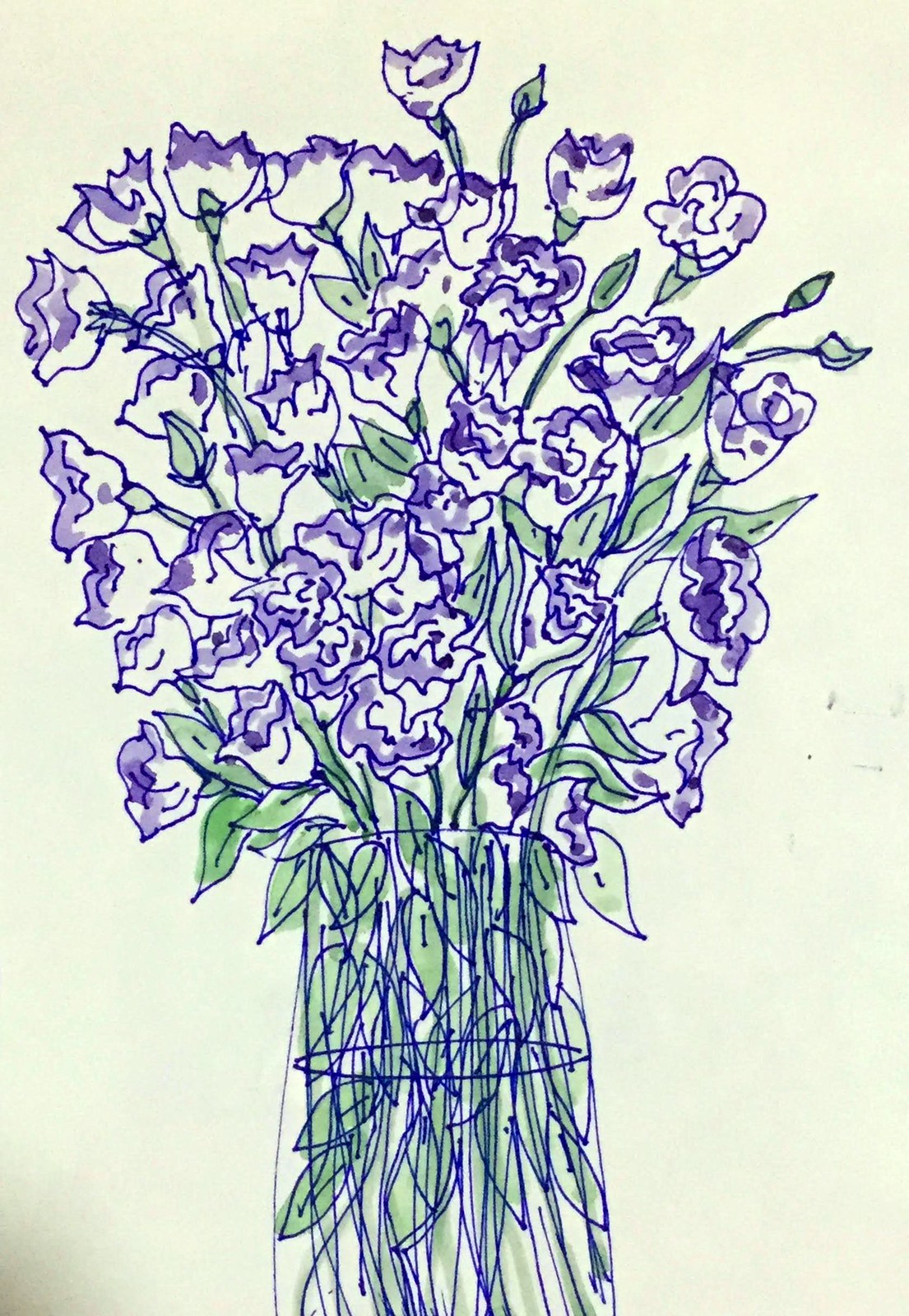This image features a charmingly primitive yet vibrant piece of artwork rendered on a vertically oriented rectangular sheet of paper. The central focus is a simple blue pen drawing of a vase, which holds a bouquet of flowers. The vase, outlined in blue ink, contains an arrangement of flowers with green stems and purple petals. The artist initially sketched the vase and flowers using the blue pen, carefully outlining both elements. Subsequently, they applied green paint to the stems and leaves, and purple paint to the blossoms, enhancing the drawing with a splash of color. The juxtaposition of the pen outlines and the painted hues creates a visually engaging piece that blends sketch and painting techniques.